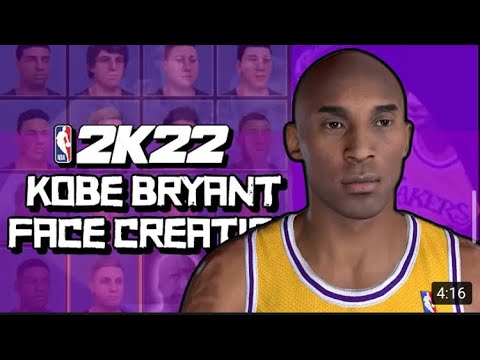This image features a screenshot from the video game "NBA 2K22" and showcases a custom-created face of Kobe Bryant. The focal point of the image is a young Kobe Bryant wearing a Los Angeles Lakers jersey, prominently displaying the NBA logo. His jersey is adorned with an emblem indicating its authenticity. There is a distinctive tattoo on his upper arm near the shoulder area, which adds to the realistic portrayal of the basketball legend. 

In the foreground, the "NBA 2K22" logo is creatively designed, with the 'O' in '2022' replaced by a 'K,' situated near the official NBA icon. The NBA logo is composed of a white silhouette of a man dribbling a basketball, with the background split into blue on the left and red on the right, with "NBA" written at the bottom. 

The upper portion of the image contains various other faces in the background against a purple backdrop, which adds depth and context to the scene, likely indicating the game's immersive environment. Additionally, the screen displays a timestamp of "4:16," hinting that this could be a still from a video segment within the game. Overall, the image captures the dynamic and intricate elements of the game's realistic representation of Kobe Bryant.